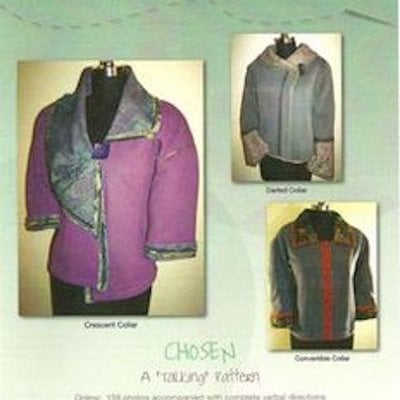The photograph appears to be a page from a pattern book advertising various sweaters and jackets. The backdrop is light green with a lighter beige section at the bottom, where text reads: "Chosen" in dark green, followed by another line in black that appears to be "tailoring pattern" but is out of focus. The image showcases three garments on black mannequins. On the left, a dark pink or light purple sweater with a large gray fur collar and mid-sleeves is displayed. In the top right, a light blue coat with light gray trim and a similar large collar is depicted. The bottom right features a darker blue coat with a red stripe down the center, brown fur collar, and cuffs. Each photograph has a beige background, emphasizing the garments' details.